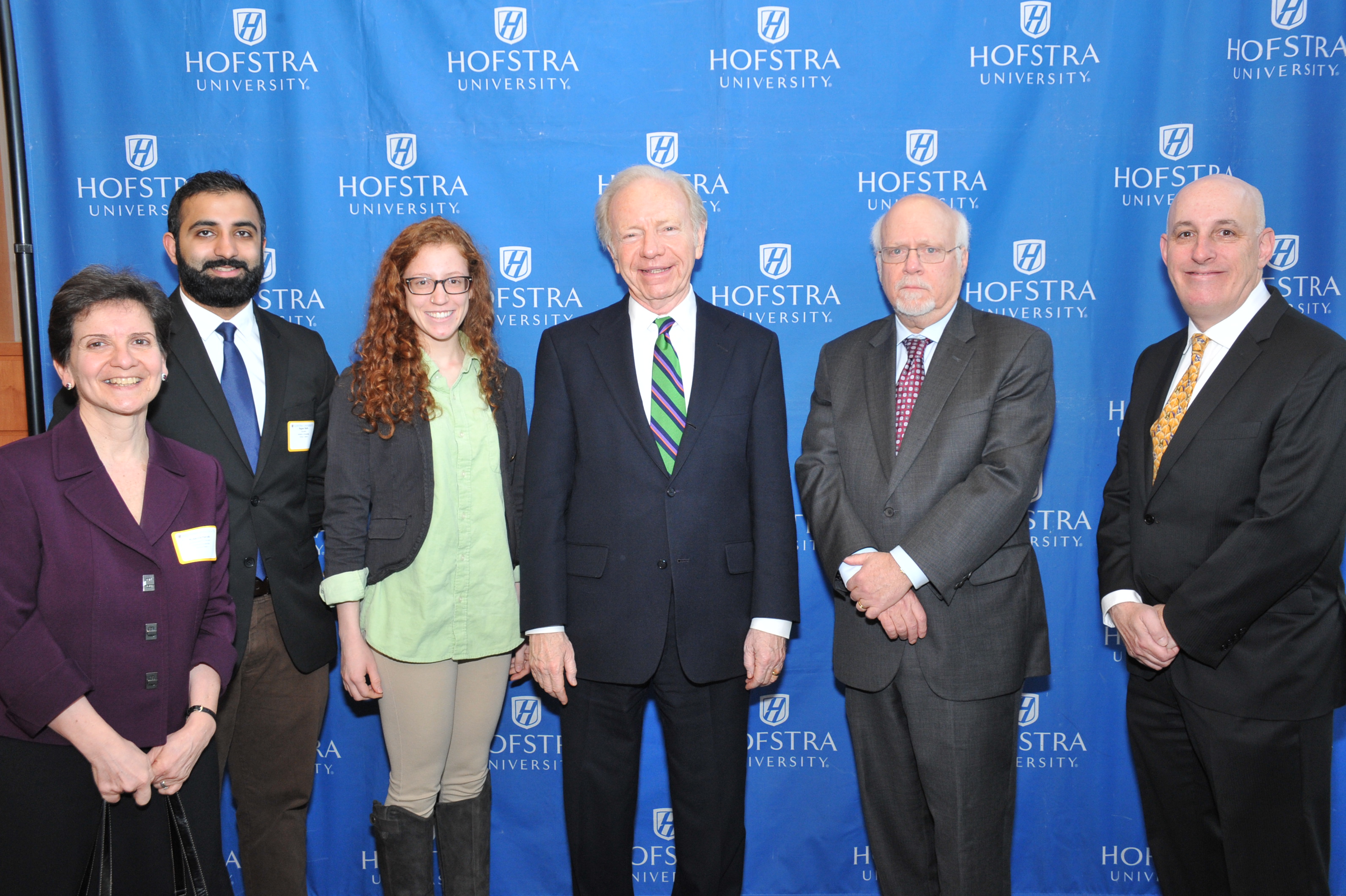In this indoor photograph set at Hofstra University, six people are posing for the camera against a backdrop featuring a repetitive blue curtain adorned with the university's logo—a white shield with an 'H' in blue, and the text "Hofstra University" written repeatedly. The background also reveals a partial view of a wooden wall to the left. Centered in the image, the group consists of four men and two women.

Starting from the left, the first woman appears to be in her 40s or 50s, wearing a purple suit jacket and black bottoms. She has short black hair and grasps a black purse with both hands. To her right is a Middle Eastern man with a thick, dark beard, short black hair, and darker skin. He sports a black suit jacket over a blue tie and white shirt, and brown pants. The third person is a younger red-haired woman, possibly in her 30s, with long curly hair and glasses. She is dressed in a dark jacket, a green top, and beige pants.

Next in line, an older man in his 60s or 70s, with white skin and smiling demeanor, wears a black suit paired with a green and purple striped tie. Beside him is another elder man with a bald head and a gray hair fringe, a gray goatee, and glasses. He dons a gray suit, conveying a serious expression. The man on the far right, likely in his 40s, has a bald head and sports a black suit with a yellow tie, completing the line-up. 

They are all framed from head to about mid-shin, with most smiling at the camera, capturing a formal yet cheerful moment at the university. The array of colors in their clothing includes brown, black, blue, white, purple, tan, light green, and pink, contributing to a dynamic yet cohesive group portrait.